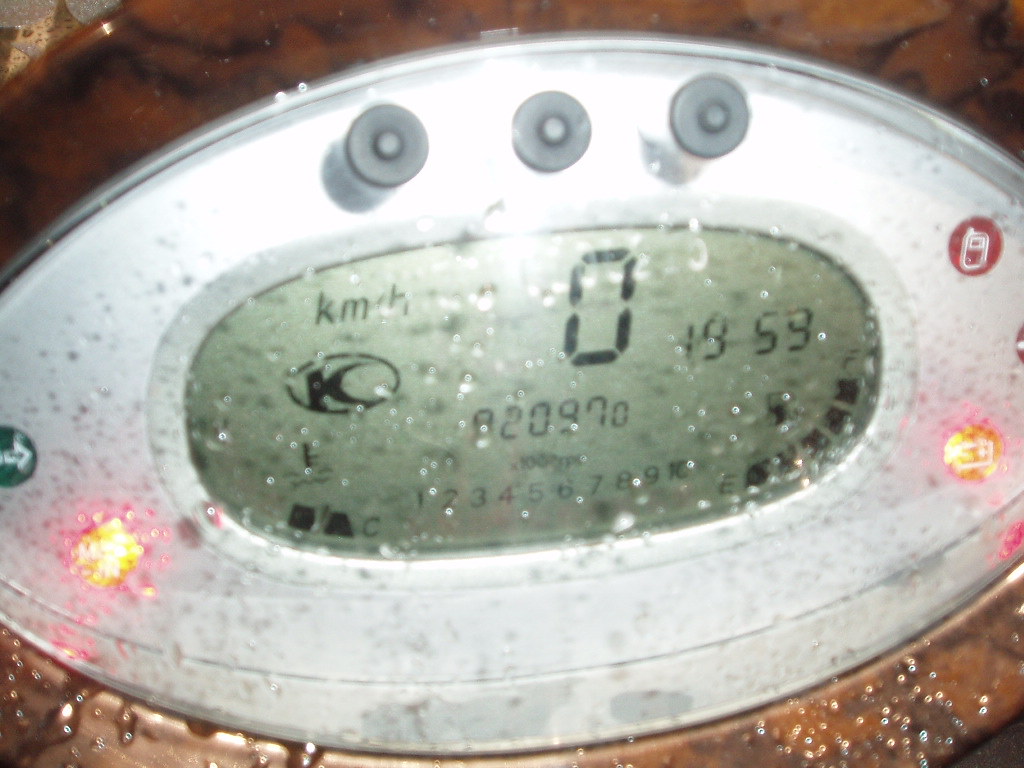This photograph captures a wet and blurry speedometer, possibly taken in the rain. The oval-shaped speedometer is predominantly silver, featuring several illuminated elements. At the base of the oval, two orange lights are visible, one on the left and one on the right. There are also a few distinctive buttons: a green bubble with a white arrow on the left, and a red circle with a white square on the right. The center of the speedometer is digital, displaying "km/h" for kilometers per hour, and it currently reads a speed of zero, indicating the vehicle is stationary. Additionally, the screen shows a time of 19:59 and an odometer reading of 2,097 kilometers. The bottom section of the speedometer face is lined with numerical indicators, partially obscured by the water droplets and blur.